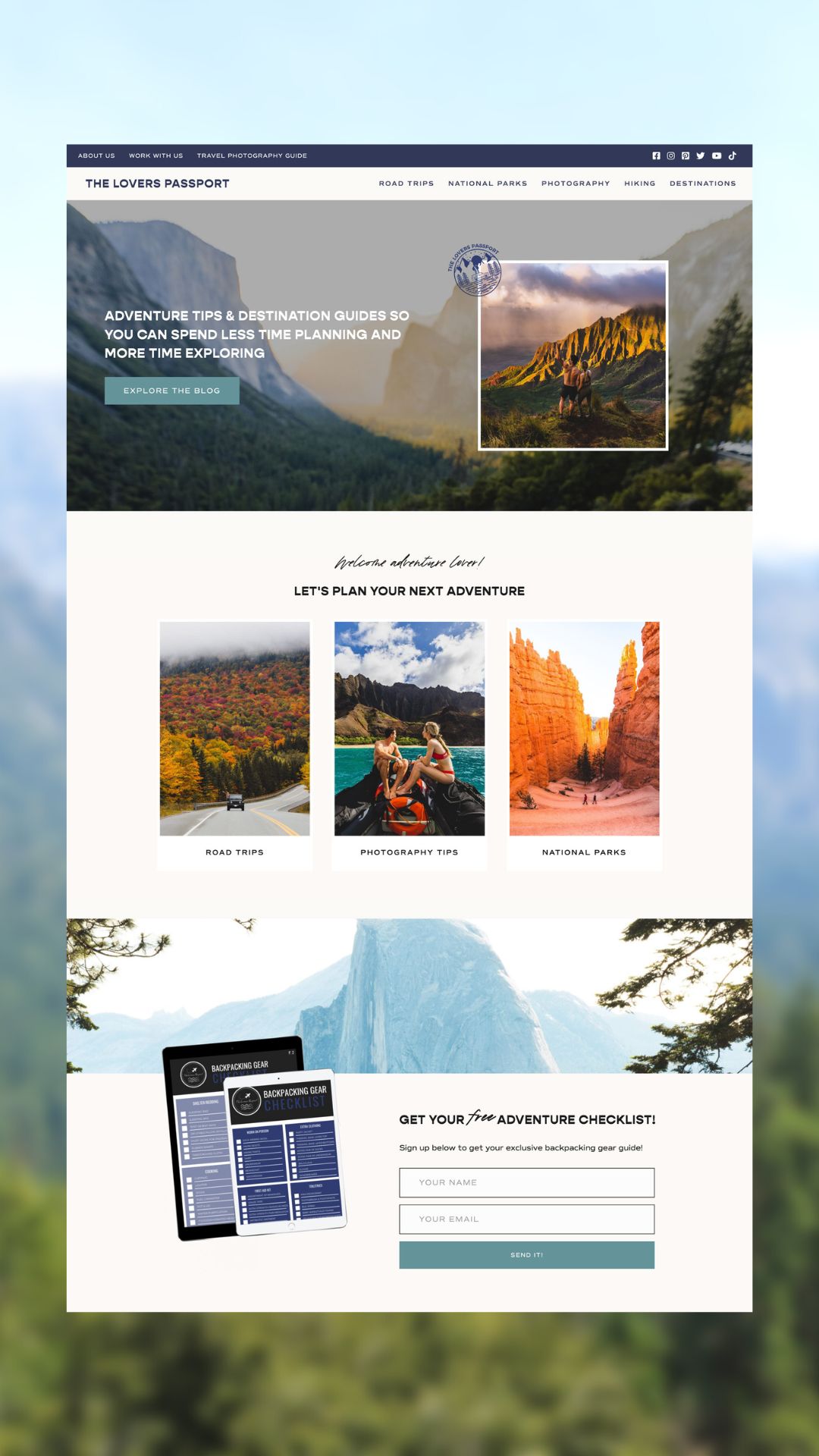In this vibrant and engaging website, titled "The Lovers Passport," we are greeted with an eye-catching and colorful design. The homepage features a white background with small tabs at the top for easy navigation. A blue banner prominently displays several social media icons, including Facebook, Instagram, and Twitter, inviting visitors to connect and follow for more content.

The page boasts a stunning panoramic mountain scene with a rich twilight sky, adorned with soft clouds. In the foreground, two adventurers stand triumphantly on a mountain range, absorbing the beauty around them. This inspiring image is complemented by the tagline in white text: "Adventure tips and destination guides so you can spend less time planning and more time exploring." A prominent blue button labeled "Explore" invites visitors to dive deeper into the site.

A central message reads, "Let's plan your next adventure," promising a helping hand in organizing future escapades. Below, a captivating photograph showcases vibrant fall foliage with a wanderer driving through the scenic landscape, accompanied by helpful guides on "Road Trips" and "Photography Tips." Additionally, another photograph captures two people sitting on a rock, gazing out at the breathtaking blue waters of the Caribbean. This site clearly aims to inspire and assist would-be travelers in discovering and enjoying their next great adventure.